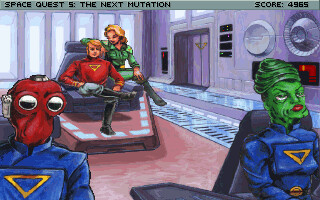The image is a colorful still shot from the video game "Space Quest 5: The Next Mutation," featuring a score of 4965 displayed at the top within a thin silver banner with black lettering. The scene unfolds on a spaceship bridge reminiscent of a Star Trek design, characterized by a pink floor and gray-purple walls adorned with large mirrors. At the center, a blonde captain in a red shirt sits in a gray captain's chair, with a buxom blonde woman in a green jumpsuit seductively lounging on the armrest, her shoulder-length wavy hair adding to the ambience.

In the foreground, there are two separated chairs, each occupied by an alien character in a blue uniform with a gold upside-down triangle emblem. The left chair hosts a Martian-like creature with red skin and big white eyes, while the right chair accommodates a green-faced woman with wrinkled features and a beehive-style hairdo. The detailed art style resembles pen and watercolor, contributing to the vivid, cartoonish feel of the image. Electronics panels and Star Trek-like doors further establish the setting as a high-tech starship.